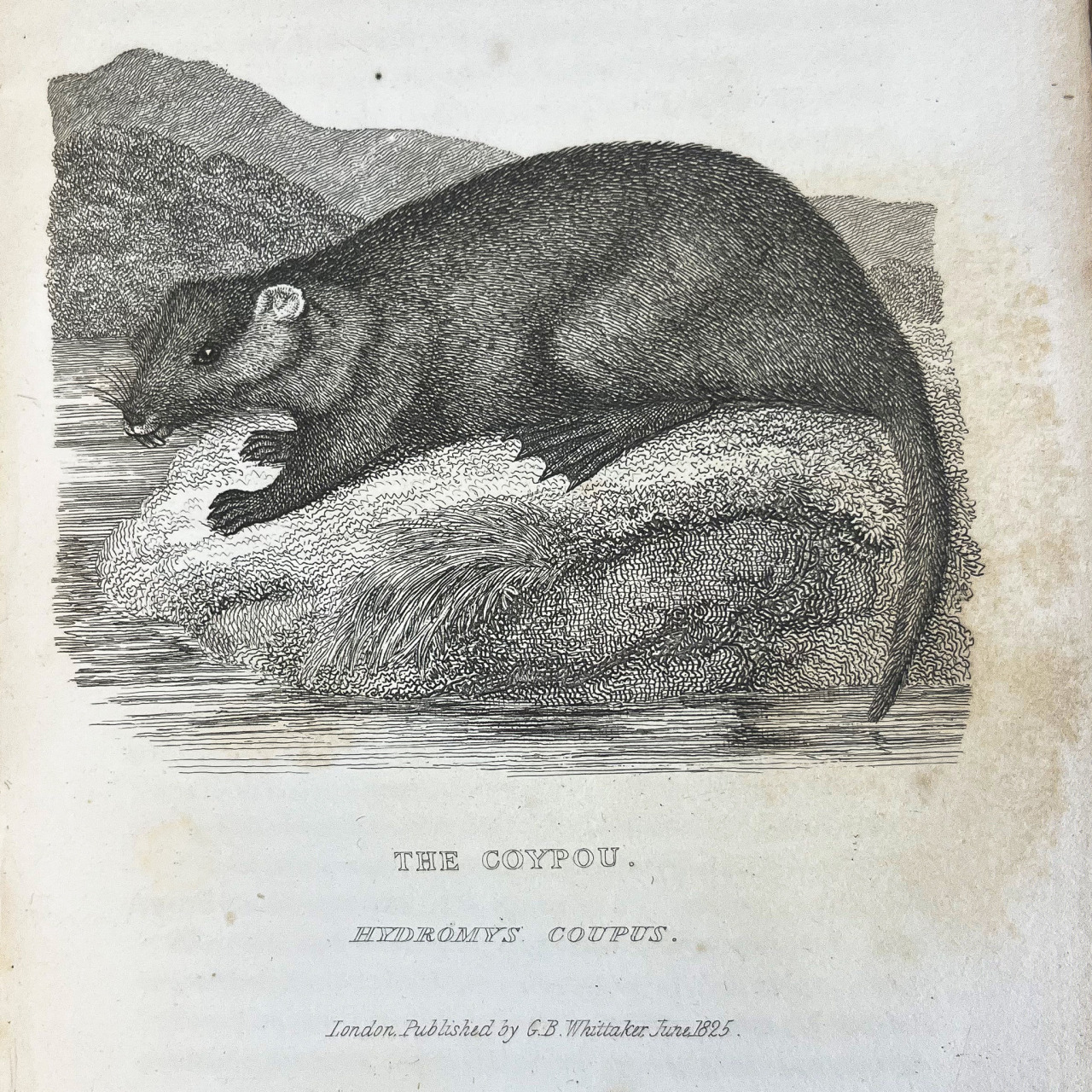The detailed black and white illustration, aged and weathered with some discoloration around the edges, depicts a creature identified as a coypu (also labeled "Hydromys Coypus" below the image). This square-shaped drawing, likely a reproduction, is centered on a rat-like animal with webbed feet, a small head with whiskers, and a furry tail. The creature is depicted sitting on a rock or mound surrounded by water, against a backdrop of hills or mountains. Beneath the illustration, in capitalized text, it reads: "THE COYPU," followed by "HYDROMYS COYPUS." Below this, it states, "London published by G. B. Whittaker, June 1825."